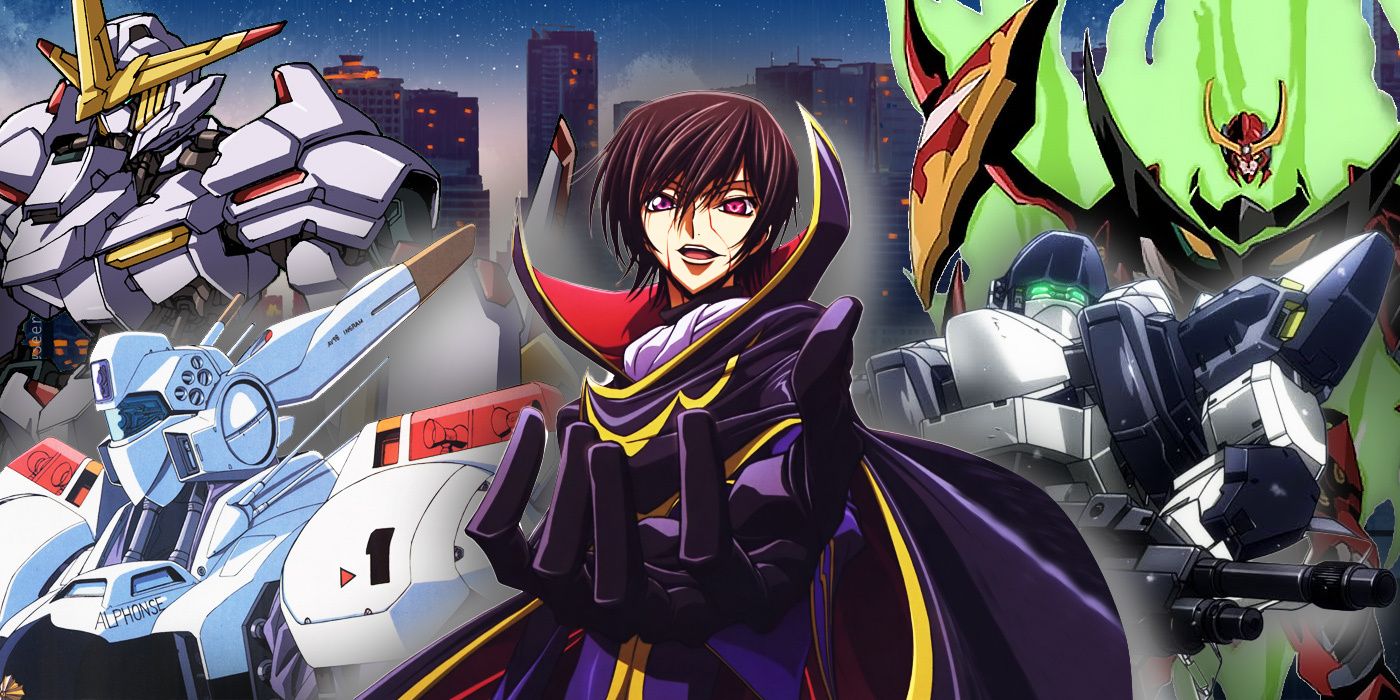The image is a digital artwork from a popular anime or manga series, specifically from Gundam. Set against a starry, dark blue sky backdrop with a cityscape featuring dark black buildings, the artwork showcases four large, distinctive robots. On the left, a bulky white robot with a yellow item on its head is situated above another white robot with red on its head. To the right, one robot is black with green elements and appears to be emitting green smoke, while another robot, characterized by its blue and white color scheme, is armed with a gun. Central to the scene is a male figure, presumably a villain, dressed in a menacing purple suit with a massive upturned collar that is red inside. He has black hair and blue eyes, and his hand is extended toward the viewer in a beckoning gesture.